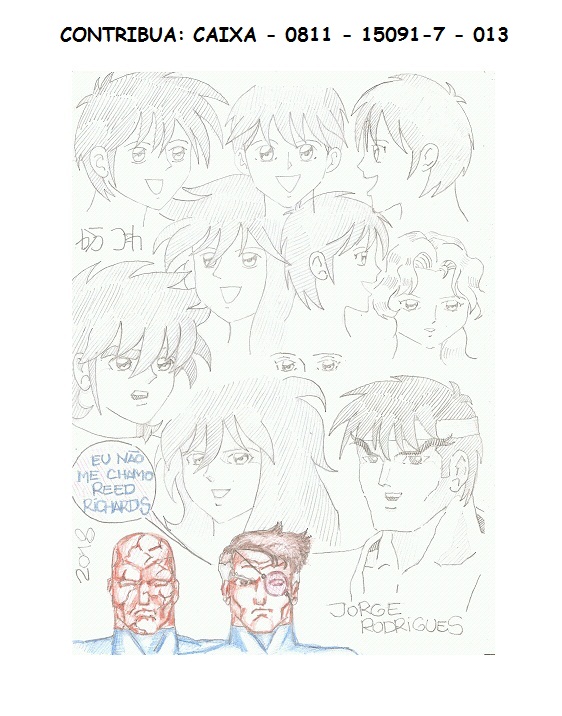The image captures a detailed collection of an artist's sketches on a white sheet of paper. The primary focus of the drawing is a series of pencil and colored pencil sketches executed in a manga comic book style, identifiable by the angular faces and large, sparkling, doll-like eyes of the characters. The sketches primarily depict male faces from various angles, including frontal and side views, showcasing figures with short, spiky hair. Interspersed among these are supporting sketches, including a girl's face with curly hair and practicing exercises such as a pair of eyes. Dominating the bottom right-hand corner are two distinct figures with colored pencil detailing: one wearing a blue top, sporting brown hair with gray streaks, and an edgy red eye patch, with a square-angled face scowling at the viewer; the second figure is characterized by a disfigured face marked with red striations, looking down with somber eyes. Above the sketches, handwritten markings "Contribua," "CAIXA," and a sequence of numbers can be seen. The signature "Jorge Rodriguez" in black letters, marks the bottom of the page, signifying the artist's completion.